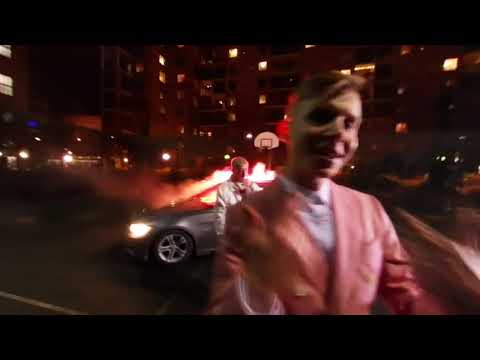In this nighttime scene, a man in his early twenties takes a blurred selfie while smiling at the camera. He wears a salmon-colored suit with a white collared shirt underneath, and has medium-length, dirty blonde hair. Behind him, another man dressed in a white suit, possibly with dirty blonde hair, stands near a silver sedan with its headlights on. The car appears to be on fire, casting an eerie light. The setting includes a basketball hoop and a large building that looks like a multi-story apartment complex, all of which suggest they are on a basketball court. The odd, chaotic scene, reminiscent of a rap music video or a movie clip, juxtaposes the formal attire of the two men with the dramatic backdrop.